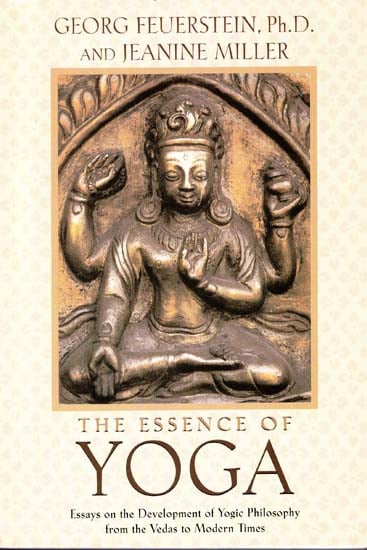This is the cover of a book titled "The Essence of Yoga: Essays on the Development of Yogic Philosophy from the Vedas to Modern Times" by George Feuerstein, Ph.D., and Jeanine Miller. The overall coloring of the cover is predominantly tan and brown with a bright, golden-bordered central image. This image depicts a brass relief of a Hindu deity in a seated, cross-legged position, adorned with a crown and earrings. The deity has four arms, each in a different posture, including one hand in front of its chest and another holding a bowl. The top of the cover features the authors' names, while the title and subtitle of the book are prominently displayed at the bottom, with "Yoga" written in a large, dark brown font.